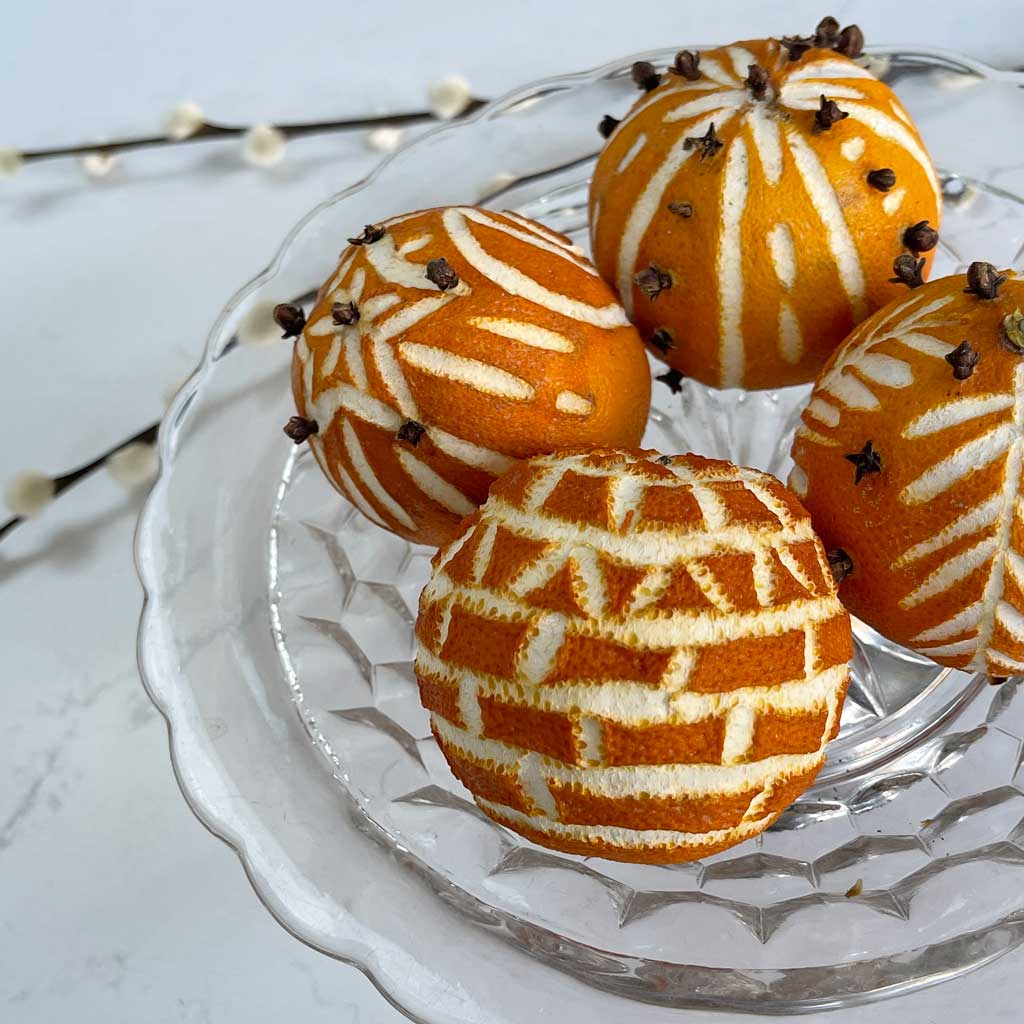This photograph captures a decorative arrangement of four oranges on a white marble countertop with subtle gray marbling. The oranges are displayed on a circular glass plate with a ridge design on the edge, and this plate is stacked on top of another circular glass plate, adding an element of depth. Behind the arrangement, two sprigs of what appear to be pussywillow branches are placed, slightly out of focus, lending a seasonal touch to the composition.

Each orange has been meticulously dried and carved with unique patterns by shaving off parts of their skins, creating designs such as bricks, stars, and leaves. These designs reveal the white pith beneath the dark orange peel, reminiscent of the sgraffito technique in pottery. Three of the four oranges also feature decorative cloves inserted into the skin, complementing the carved patterns. The cloves are arranged in various ways, such as along the lines of the carvings or highlighting specific design elements. Notably, three of the oranges also have small, brownish, and wilted buds emerging from them. One orange is partially outside the image frame, contributing to the dynamic arrangement on the pristine marble surface.